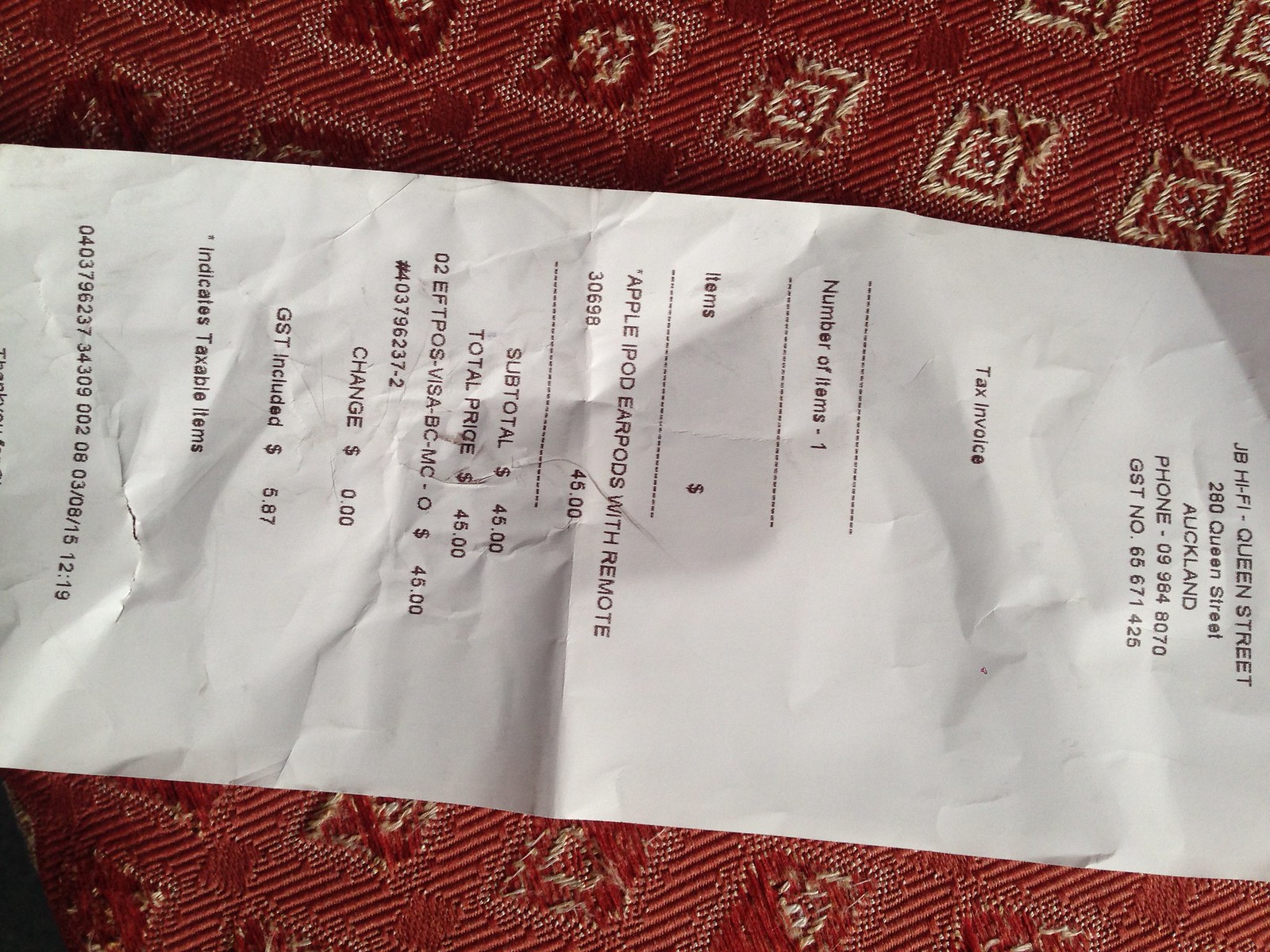The image captures a crinkled receipt laying sideways on a red tablecloth with a textured pattern, featuring beige squares with red accents. The white rectangular receipt, viewed horizontally, displays black text. At the top, it reads "JB High Pie, Queen Street," followed by the address "280 Queen Street, Auckland," a phone number, and additional identification numbers. The receipt itemizes a single purchase: "Apple iPod EarPods with remote," priced at $45. Detailed breakdowns include an item code "30696," subtotal "$45," total price "$45," with GST tax included at "$587." The bottom edge of the receipt is partially obscured, cutting off some text.